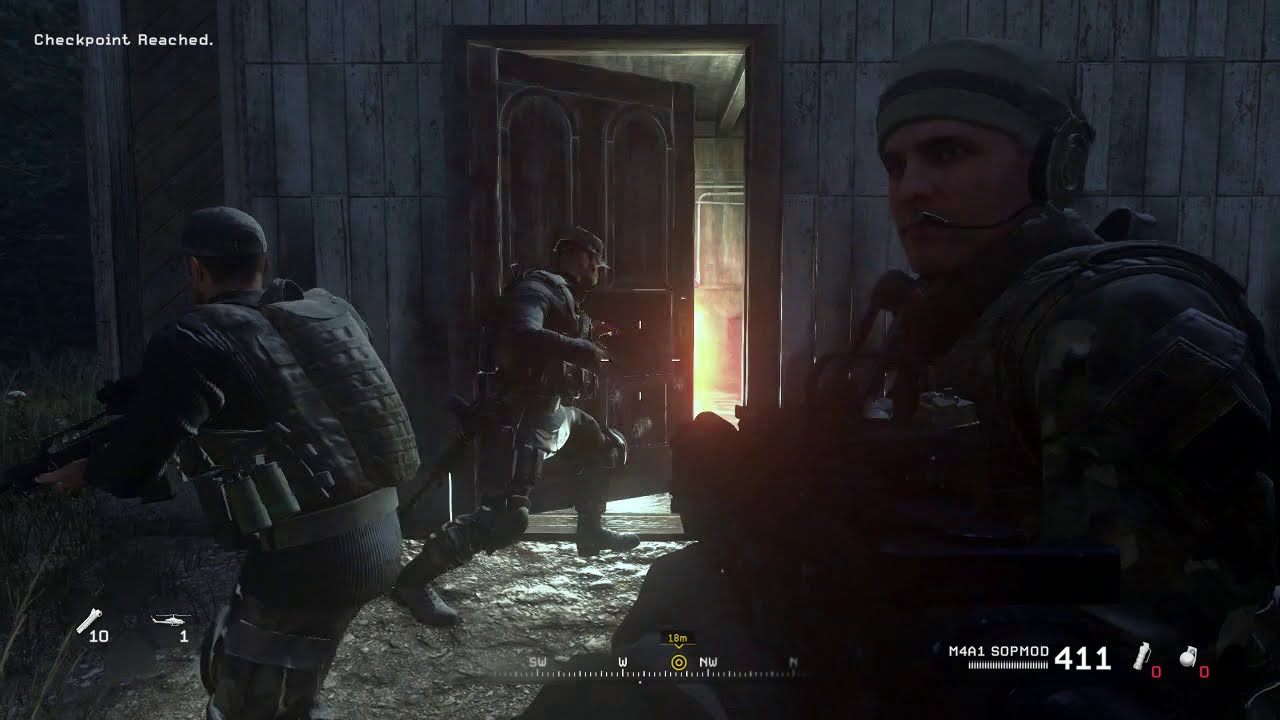The picture is a detailed screenshot from a military video game, likely from the campaign mode of Call of Duty. The scene is set in a dark and shadowy environment, possibly inside an abandoned building with a stone floor, accentuating the realism of the game. Three male soldiers clad in dark, army green tactical gear and camouflage are featured. The central soldier, facing partially away and turned to the left, strides quickly towards a door that is opening outward, revealing a bright light beyond. He has a rifle attached to his right side, suggesting imminent action. To the left, another soldier, slightly turned away, is identifiable by the caption above him reading, "Checkpoint Reached." This soldier wears a cap and a vest-like gear with various items attached, including a rifle pointed down. He’s seen alongside a white object marked with the number 10, next to a tiny white helicopter labeled with the number 1, indicating inventory tracking. The final soldier, positioned to the right, is partially turned left, revealing his headset with a microphone, signaling communication readiness. He also dons a cap and has dark eyebrows and eyes, with gear similar to his comrades. Below him, white text reads "M4A1 SOP MOD 411," detailing his weapon and ammunition count. The screen further shows a compass at the bottom center, displaying directional markers "SW, W, and NW," assisting gameplay navigation.